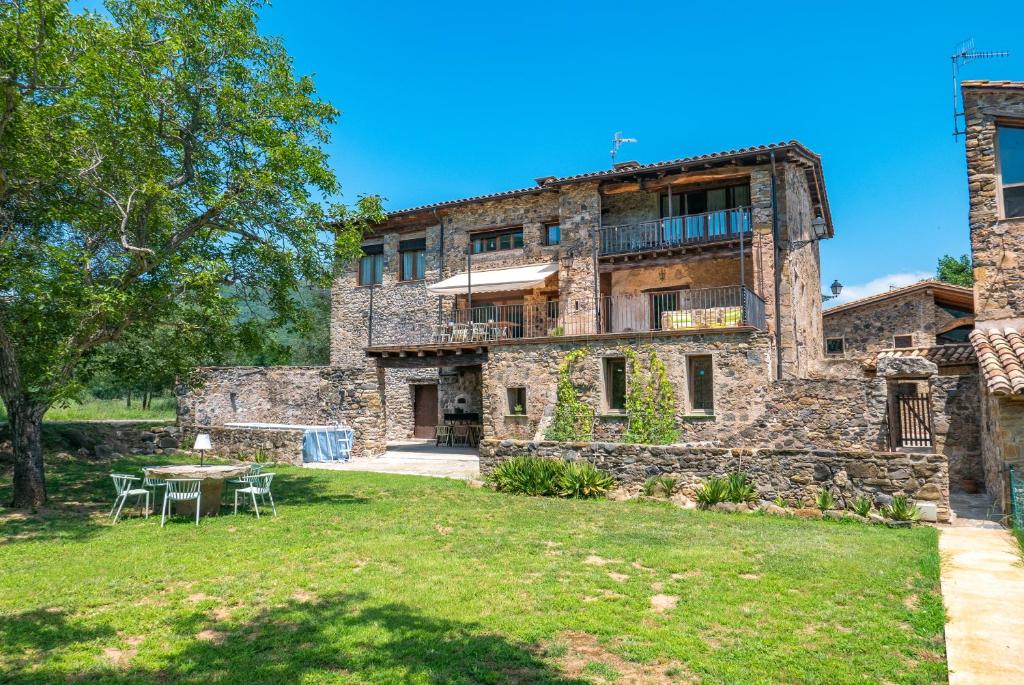This landscape-oriented photograph captures a sprawling, three-level stone house with a light brown to tan hue. The house stands majestically behind a grassy yard, which takes up the lower third of the image. The yard features some brown blotchy spots, hinting at a hot climate or irregular lawn maintenance. A paved, light brown concrete walkway extends from the bottom right corner towards the house. Just off the walkway, a table and several white chairs are positioned on the lawn, with a white lamp placed on the table, suggesting an inviting outdoor seating area. 

In the upper left corner of the image, a large green tree with pointy leaves adds a touch of nature against the clear blue sky, which has no clouds. The house itself showcases a robust structure with numerous stone blocks comprising its foundation. 

On the right side of the house, there is a wooden front door on the ground floor, along with three visible windows. The second level features a balcony and an awning, with glass doors that open onto the deck, which is enclosed by metal railings. The roof has a trapezoidal shape, and an antenna is installed on top, implying antenna-based television reception. The photograph cuts off part of the house on the right and left sides, giving only a partial view of its full expanse. In this serene setting, the combination of natural and built elements creates a picturesque and inviting scene.